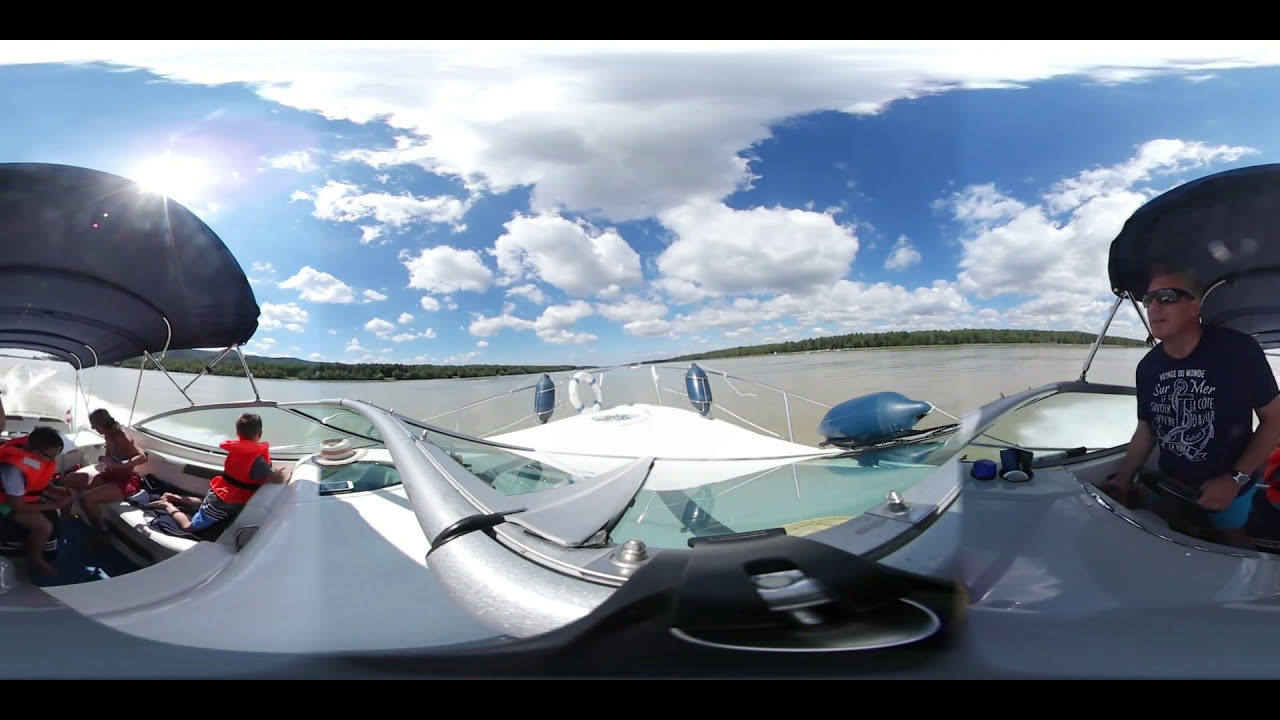The image is a 360-degree panoramic shot taken on a boat on a river or lake, capturing a full view from the front to the back of the boat. On the far right, the older driver is slightly leaning forward, one hand on the wheel and the other on control paddles beside him. He's wearing sunglasses, a blue t-shirt adorned with white writing down the center, and a watch on his wrist. Above him is a gray, round canopy providing partial shade.

In the left part of the image, three people are sitting. Two of them, including a small boy, are wearing orange life jackets. The child is on his knees, leaning against the side of the boat, peering out through a window. Another person behind him, also wearing a life jacket and sunglasses, is slouched with arms in front, looking downward. The third person seated near the back, wearing shorts without a life jacket, also appears to be looking down. Around the midsection of the boat are metal railings and plastic cylinders or capsules hanging on the sides.

Surrounding the vessel is brown water, bordered by greenery and trees on either side. The sky above is a clear, vibrant blue, adorned with white clouds and the sun prominently positioned in the top left corner, illuminating the scene. The entire boat, with its white body, is fully visible in the shot, encapsulating a serene, sunlit day outdoors.